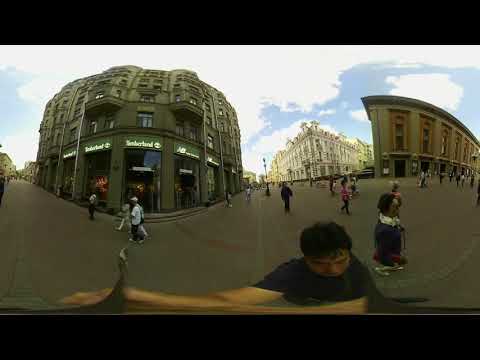The image is a 360-degree panoramic shot taken in a downtown area on a cloudy day. The scene is dominated by a stone pavement in the forefront, where a few people are scattered, walking and possibly shopping. The background reveals a mix of buildings, including a white corner building on the right that extends horizontally and other commercial structures with various storefronts on the lower levels. A notable feature is a tall white building several stories high, positioned against a light blue sky with clouds. The setting is daytime, with no vehicles in sight, and the elements in the image, including colors like black, white, gray, blue, green, tan, red, and yellow, appear slightly distorted due to the wide-angle effect of the panoramic shot. A man in the foreground, holding something, is likely the one taking the photo, which explains the warped perspective of the surroundings.